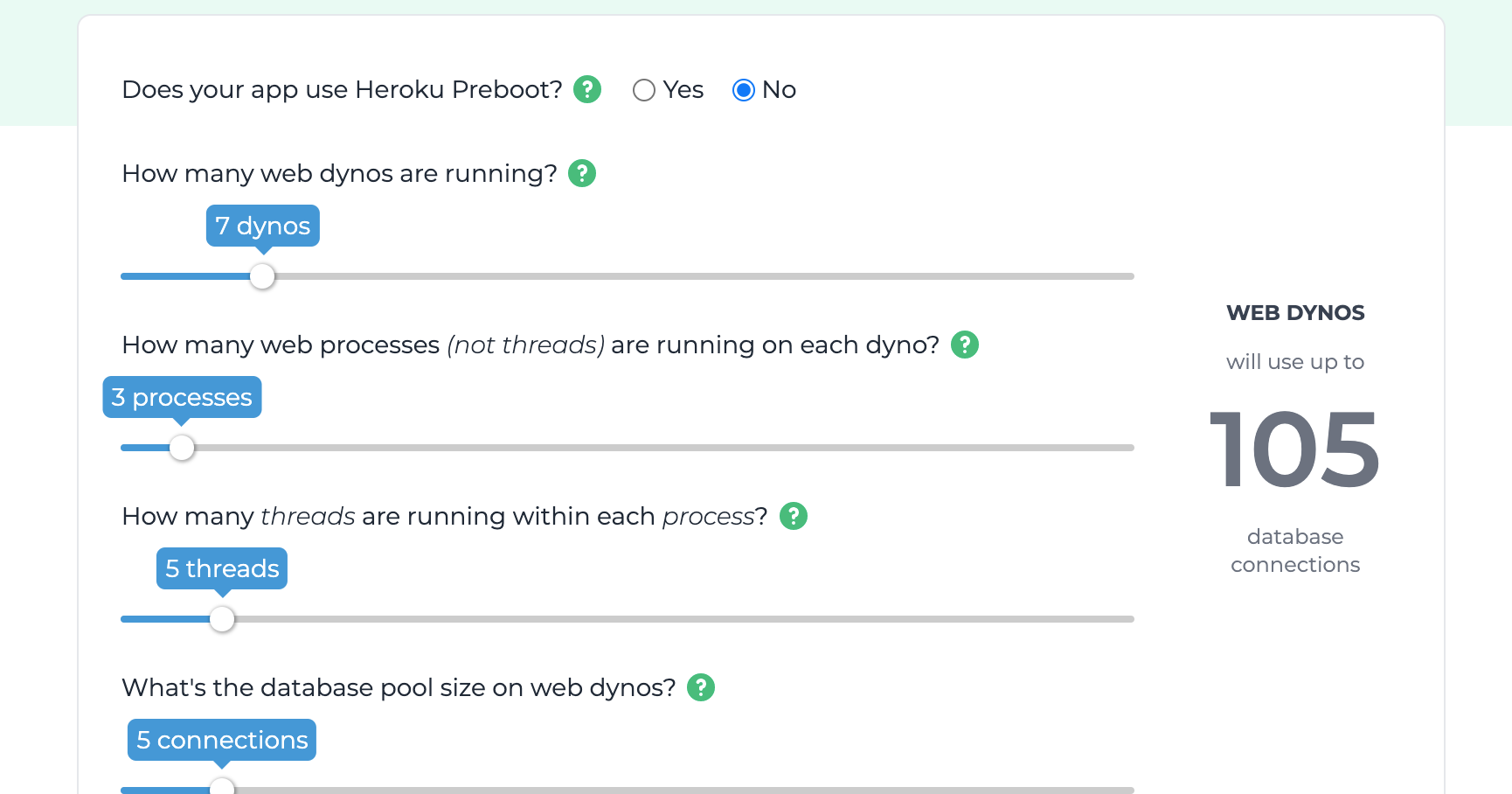The image showcases a screenshot of a web dashboard providing an overview of the configuration settings for a Heroku app's web processes.

At the top, the title reads: "Does your app use Heroku (H-E-R-O-K-U) Reboot?" Below this title, there’s a green circle with a white question mark symbol, indicating an information or help icon. Adjacent to this, there are two options: "Yes" and "No", displayed as clickable radio buttons. The "No" option is selected and highlighted in blue.

Next, the section asks, "How many web dinos are running?" accompanied again by a green question-mark icon. Below this query lies a slider bar. The bar is set significantly to the left, showing a small blue segment and a larger gray segment, indicating the proportion of the setting chosen. A blue bubble displays "7 dinos" in white text.

Following this, the section inquires, "How many web processes, not threads, are running on each dino?" Alongside this, the standard green question-mark icon is present. The corresponding slider is also placed to the left, with minimal blue compared to the gray area. A blue bubble displays "3 processes."

Further down, the slider asks, "How many threads are running within each process?" The green question-mark icon stands beside this query. Its accompanying slider is positioned more to the left, with gray dominating the bar. A blue bubble shows "5 threads" in white text.

Lastly, the dashboard reviews, "What's the database pool size on the web dinos?" with the familiar green question-mark icon. Below lies another slider, mostly gray with a small blue segment. Inside a blue bubble, "5 connections" is written in white text.

On the right side of the image, there’s a summarized note stating: "Web dinos will use up to 105 database connections."